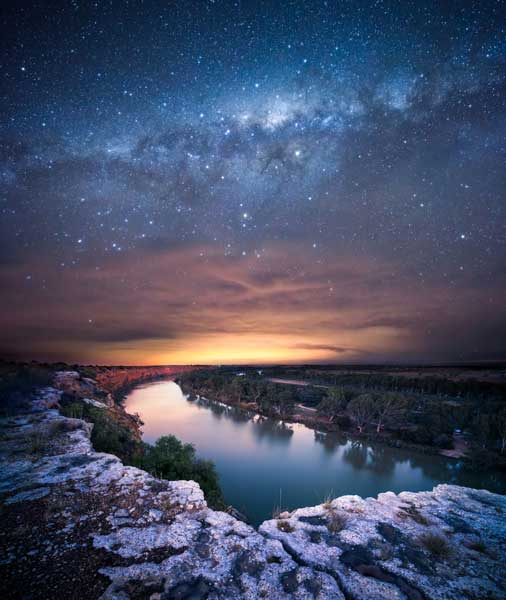The image is a vertically rectangular, full-color photograph taken near twilight, likely digitally enhanced to emphasize its celestial elements. The top two-thirds of the image is dominated by a captivating night sky, displaying an exceptionally pronounced Milky Way filled with an abundance of stars, much clearer and more vibrant than usually visible to the naked eye. The horizon glows with the orange and yellow hues of a setting or rising sun, transitioning into soft pinks and purples, and finally deepening into a rich blue with the stars becoming sparser but still prominently visible. Below this stunning sky, a tranquil river or lake curves gracefully through the scene, beginning at the bottom right and arching towards the center before curving back left. The body of water, reflecting the encircling green trees, appears blue-green and extremely still. The foreground of the image features a rocky gray plateau that offers a vantage point from which the river or lake is viewed, adding a rugged texture to the serene landscape. The left side of the river is flanked by a high ridge lined with dense greenery, while the opposite side showcases a lower, tree-lined shore. The entire composition, bordered by natural elements, creates a harmonious blend of land, water, and sky, offering a breathtaking view of nature under a star-studded night.